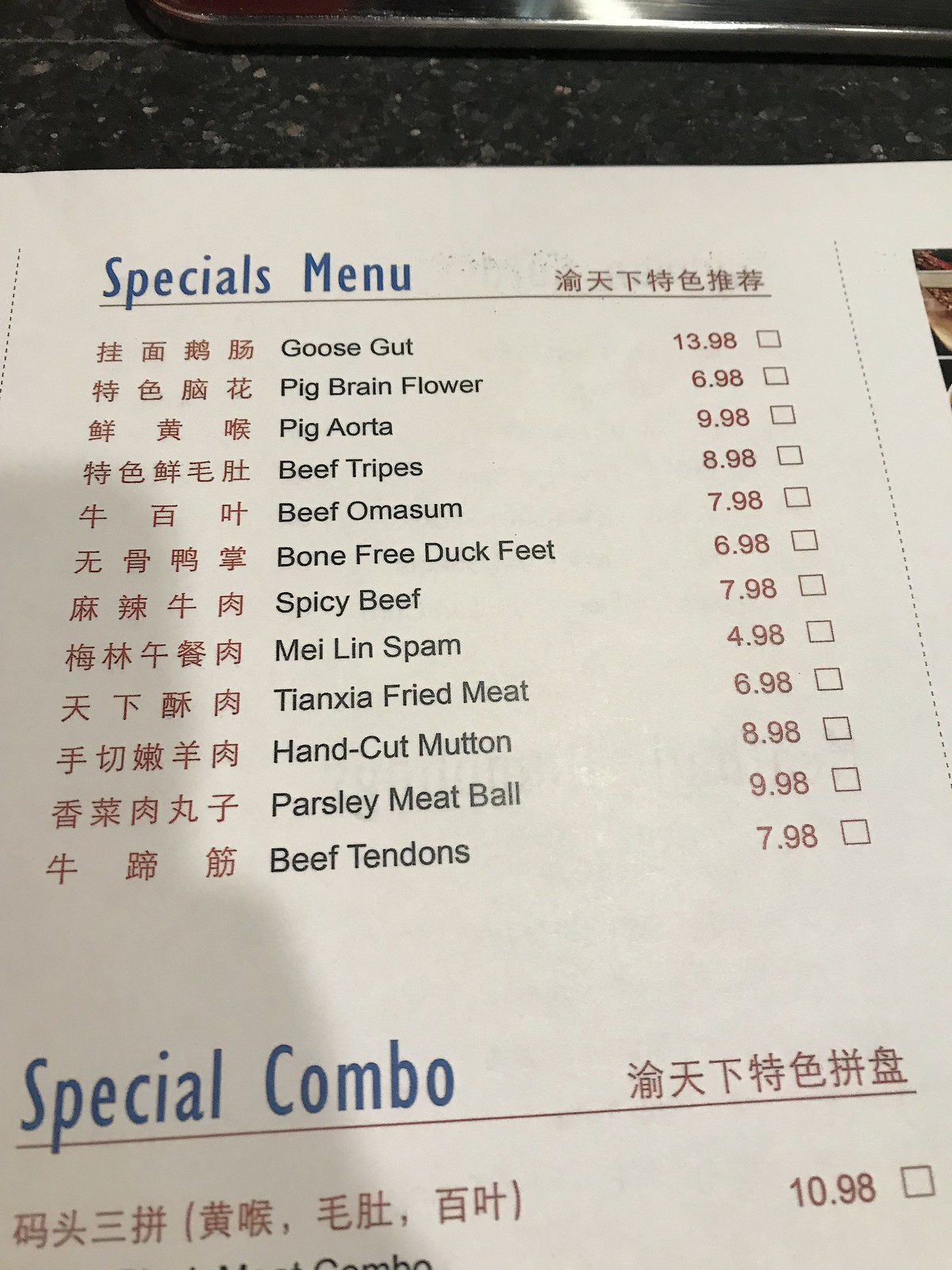The image showcases a specials menu at an Asian restaurant. At the top of the menu, "Specials Menu" is prominently displayed in blue, accompanied by Asian characters in a reddish-orange hue to the right. Below, the menu features a list of dishes, each presented with Asian characters followed by their English translation in black and the corresponding price in red. The dishes and their prices are as follows:

- Goose Gut: $13.98
- Pig Brain Flour: $6.98
- Pig Aorta: $9.98
- Beef Tripes: $8.98
- Beef Omasum: $7.98
- Bone-Free Duck Feet: $6.98
- Spicy Beef: $7.98
- Mei Lin Spam: $4.98
- Tian Jia Fried Meat: $6.98
- Hand Cut Mutton: $8.98
- Parsley Meatball: $9.98
- Beef Tendons: $7.98

Adjacent to each price, there are empty squares, likely for selection or quantity notation. At the bottom of the menu in blue lettering, "Special Combo" is noted, again featuring similar Asian characters. The special combo is priced at $10.98, though part of the word "combo" is truncated in the image.